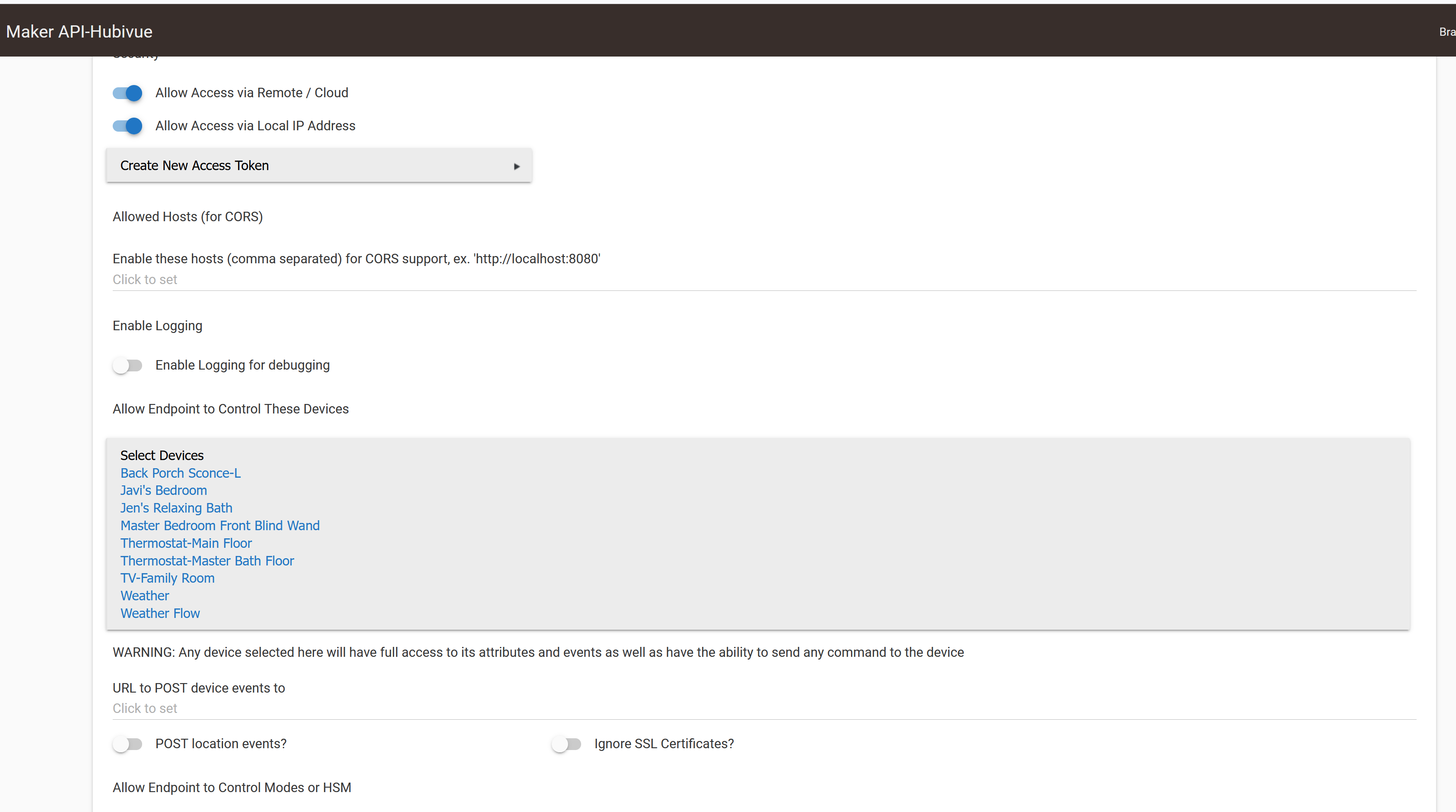The image depicts a website interface with a detailed configuration screen. At the top, there is a black header featuring small white text in the top left corner. Below this header, two options are present, both toggled on with blue buttons. 

Following this, a gray rectangle occupies the space, containing centered black text. Beneath this rectangle, more black text appears followed by a horizontal divider line stretching from one side to the other.

Next, the phrase "Enable Logging" is displayed with a toggle switch set to off. Below it, another setting reads "Allow endpoint to control these devices," leading into a gray subsection.

This gray subsection, which spans the width of the screen, states "Select Device" and lists nine selectable options in small blue text. Below this list, a warning label is present.

Further down, the screen displays "URL to post device events to" with an accompanying text field. Next, the option "Post location events?" is shown with a toggle switch set to off, followed by "Ignore SSL certificates," also toggled off.

Finally, at the very bottom, the text reads "Allow endpoints to control modes," concluding the configuration options depicted in the image.